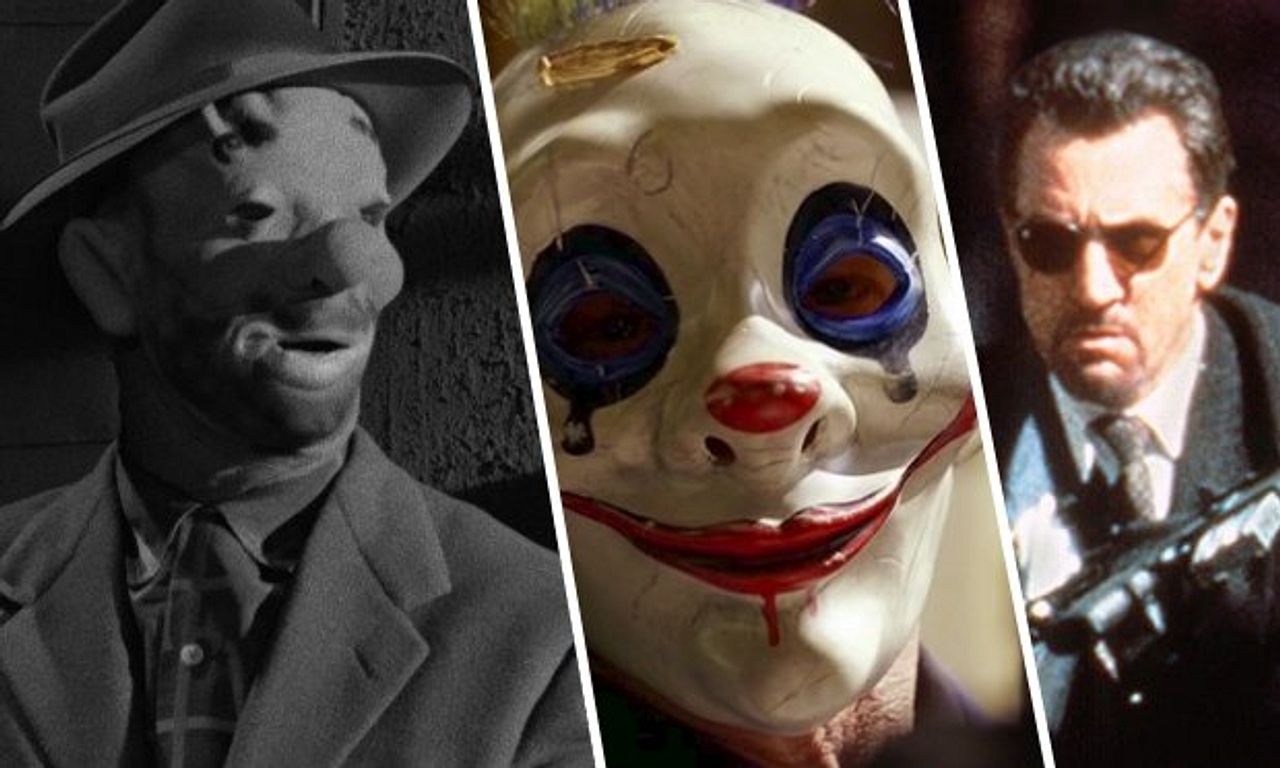This image is a wide, rectangular collage separated by thick white diagonal lines, organizing three distinct portrayals. The left section, being the largest, is a black and white photograph of a man in a clown mask. He sports a plaid dark shirt under a gray wool coat and a fedora, providing a vintage feel. The mask, characterized by a large clown nose and distorted ears, lends an eerie ambiance while he gazes diagonally to the right. In the center, a vivid, colorful close-up depicts another man in a clown mask reminiscent of a character from the movie "It." The shiny white mask features blue accents around the eyes, a red circle on the nose, and red lips adorned with what seems to be blood. Lastly, the rightmost image showcases a man resembling Robert De Niro. He has dark brown hair, wears sunglasses, and sports a goatee. Holding a camera around his neck, he exudes a sense of intensity, contributing to the collage's overall dramatic theme.